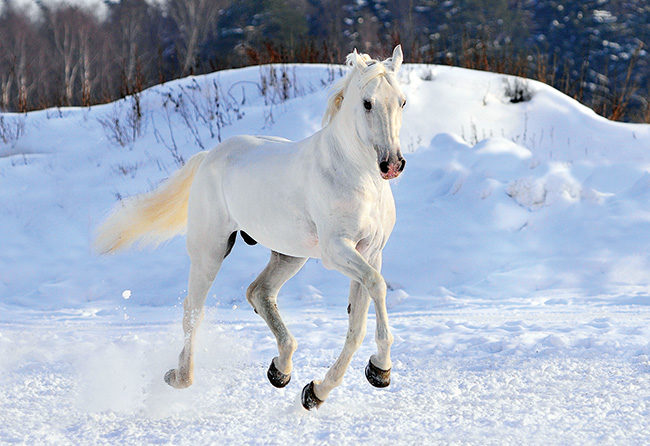A stunning and captivating image showcases a striking, all-white horse galloping gracefully through a snowy wilderness. Captured mid-trot, the horse is completely airborne, its black hooves off the ground as it surges forward. The scene is set outdoors in a wintry landscape, with a clear sky indicating a bright, sunlit day. The horse's white fur gleams against the fluffy, thick snow, and its mane and tail, tinged with a light yellow hue, flow beautifully as it runs. The snout is black with a subtle pink center, and the horse's dark, expressive eyes contrast with its white coat. A plume of snow is stirred up behind its hind legs, emphasizing the speed and power of its motion. Surrounding the horse is a snowy surface, where a rising snowbank dotted with leafless twigs extends into the distance. Beyond this, various tree trunks, some possibly pine, stand bare, adding to the stark beauty of the winter scene.